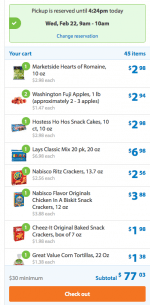The image is a screenshot of a cell phone app, which could also be a website, and is tall and narrow, approximately three times as high as it is wide. At the top of the screenshot is a green rectangle featuring a lighter green interior with centered black text indicating a reserved pickup time: "Pickup is reserved until 4:24 PM today." Just below this, additional text states, "Wednesday, February 22nd, 9 AM to 10 AM." A blue link below this text reads "Change reservation" and includes a green check mark on its left side.

Outside this green area, to the left, blue text reads "Your cart," while on the right, "45 items" is displayed. The cart itself features a vertically scrolling list, currently showing images and prices of eight grocery items, though the last item is partially cut off, indicating more items below. The item prices are prominently displayed in blue on the right side of the screen.

At the bottom of the screenshot, a separate section with a light blue background declares a "$30 minimum" order requirement, while the right-hand side of this section shows "Subtotal" in blue text next to a large subtotal amount of $37.03. Finally, at the bottom of this section, a large orange button with white text in the center reads "Checkout."